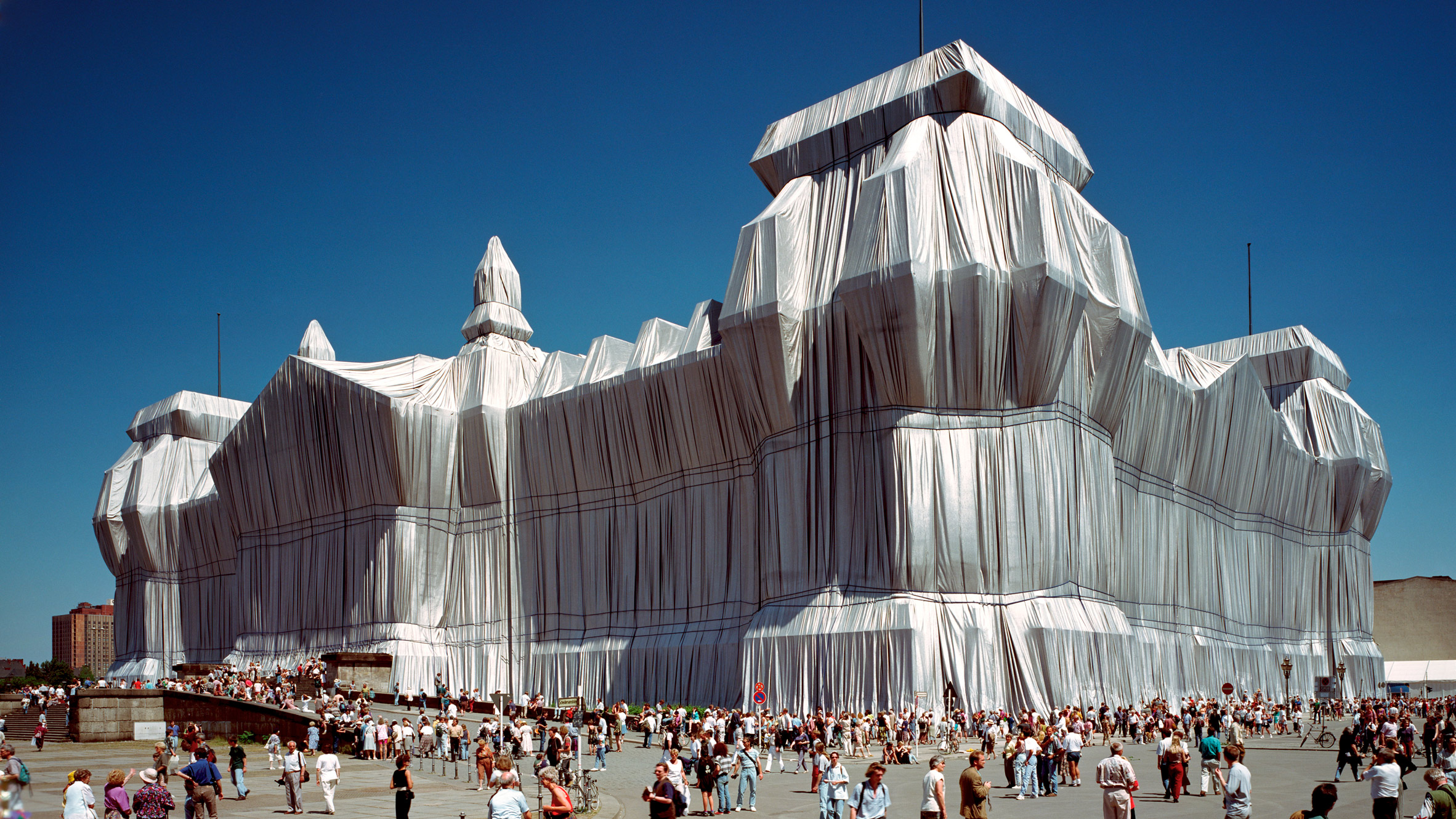In this vibrant city center photograph, a towering, multi-leveled structure, potentially a cathedral or mausoleum, stands prominently draped in large silver curtains, reminiscent of Christo's artwork. The draped sections conceal much of the old, stone architecture beneath, save for a few spiked tops peeking through. Surrounding the structure, hundreds of tourists in multicolored shirts—blue, white, brown, pink, purple, and black—mill about, snapping photos and absorbing the scene on this sunny day. The sky above fades from a deep blue at the top to a lighter blue near the horizon, accentuating the structure's silvery shroud. In the distance, modern buildings punctuate the skyline, contrasting with the historical feel of the covered building. Hills and mountains faintly trace the background, completing this lively tourist hub.